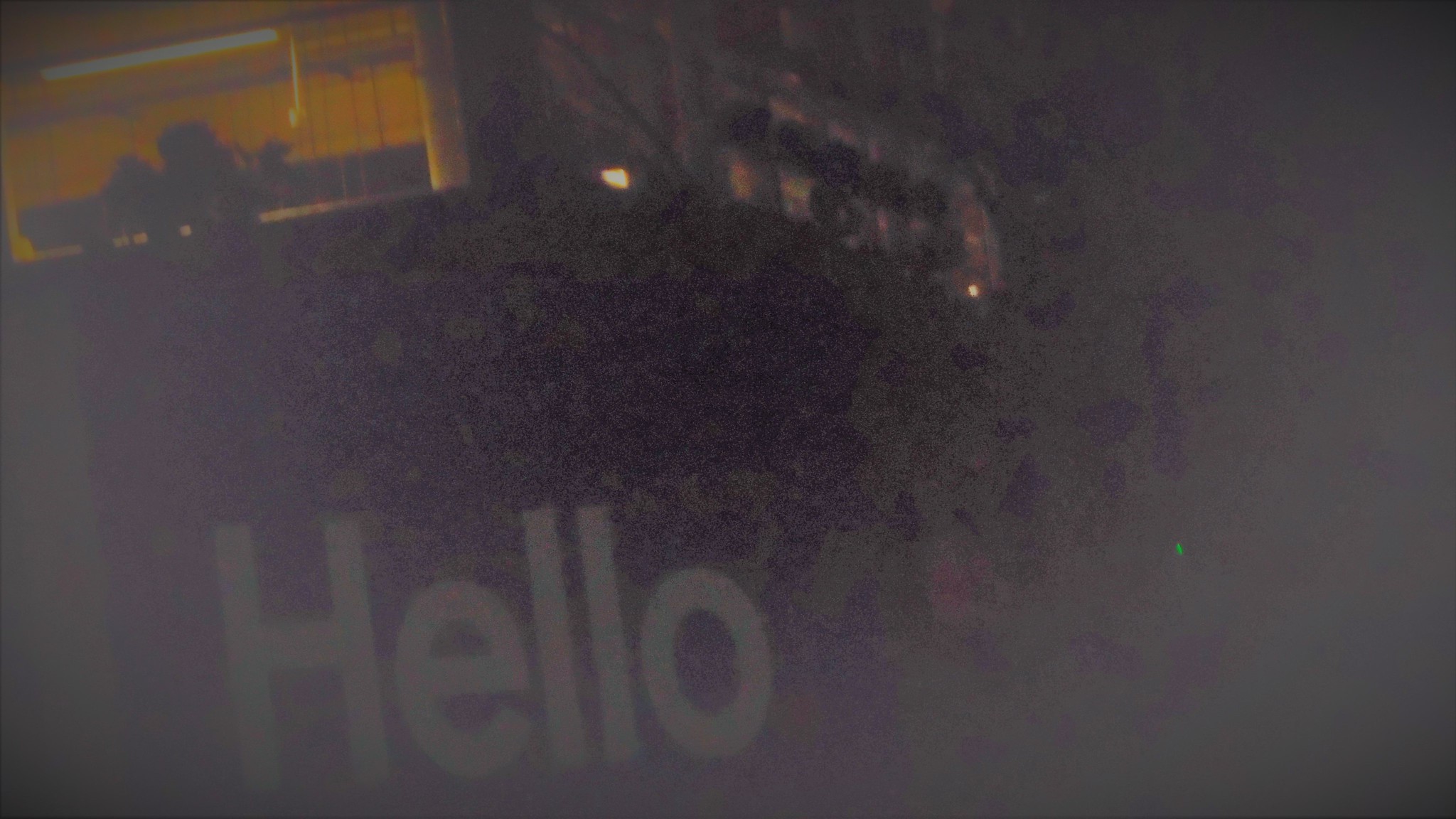A dark, outdoor scene featuring a black sign with the word "HELLO" written in bold white letters. In the background, there appears to be a window, possibly from an apartment building or campus housing, with some other lights faintly visible. The overall lack of illumination makes much of the image obscure, though one distinctive green light stands out. Tree branches and various outdoor elements are faintly visible, suggesting the setting is outside. Amidst the dim background, an orange-hued light, reminiscent of what you might find in a classroom or large room, adds a splash of color to the scene.